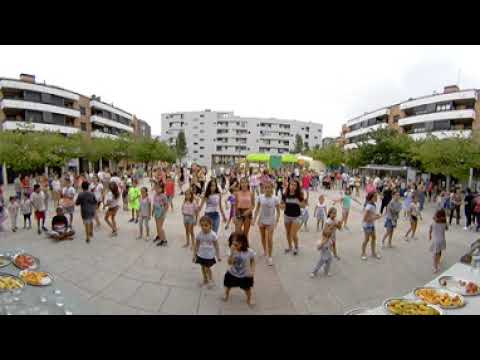In this wide-angle photograph of a bustling town square, the scene captures what appears to be a lively party, possibly a communal celebration. The plaza, a round cement area, is filled with a diverse group of people, highlighted by a multitude of children at the forefront facing the camera, seemingly engaged in a coordinated dance. The children are joined by several adults and older children standing behind them. 

To the right of the image, there’s a long white table laden with an assortment of food, possibly including plates of pizza and other dishes, giving the impression of a festive feast. A similar table with more food is partially visible on the left side of the image. The background reveals various structures; to the right and left, there are brick office buildings with distinct white visors above the windows, each sporting flat-top roofs. These buildings are approximately three stories high. 

Further back, a taller, white building with many windows rises, potentially a housing complex or hotel, approximately six stories tall with balconies. The plaza is dotted with trees, and a green pavilion can be seen towards the edge. The sky is markedly white and overexposed, suggesting a cloudy day without distinguishable clouds.

The overall atmosphere is one of community and togetherness, underscored by the uniformity of many attendees wearing white t-shirts. The entire composition, framed by black stripes at the top and bottom, emphasizes the depth and expanse of this festive gathering.